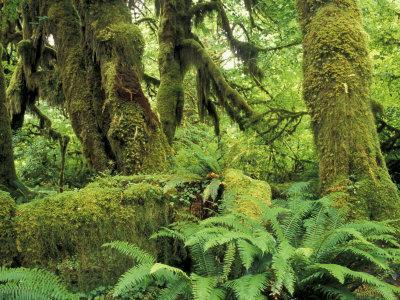This image presents a dense, lush jungle setting captured in a slightly blurred photograph. The backdrop of the image is filled with a vibrant array of greenery composed mainly of trees cloaked in verdant moss. Moving closer in the frame, the photograph showcases several large tree trunks, one particularly notable for its distinctive U-shaped arch, all enveloped in rich, greenish-brown moss. The foreground is dominated by sprawling, bright green ferns, their leaves extending outward with a subtle yellow tinge, standing tall amidst the moss-carpeted undergrowth. Above, a thick canopy of leaves interlaces to allow only slivers of sky to peek through, creating a rich tapestry of various green hues. Despite the sheer abundance of vegetation, there are no visible signs of wildlife or humans in this tranquil, plant-dominated scene.